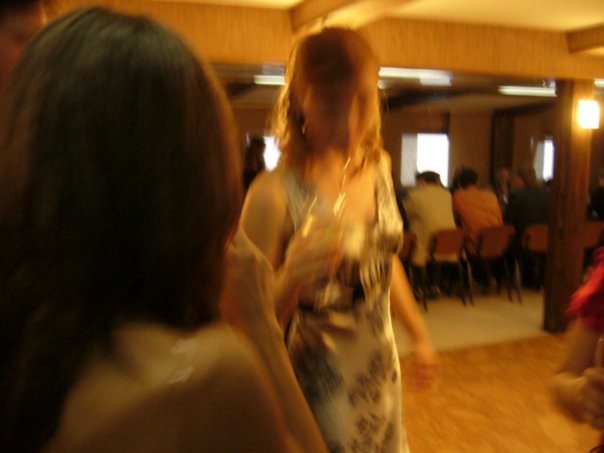In a room with high, vaulted ceilings showcasing a light-colored ceiling and intricately exposed wood framework, people have gathered. The wooden framework, supported by medium-toned wood pillars with visible grain, offers an elegant and rustic touch. At the center of the image, albeit blurred, stands a woman dressed in a silver, floral-patterned dress, possibly with darker flowers such as purple. She holds a long-stemmed glass containing what appears to be amber-colored liquid, perhaps a cocktail or wine. The back of another woman with long, dark hair and glistening skin, possibly adorned with a strap is visible, indicating she might be wearing a shimmering garment. Seated around what seems to be a bar area, though not clearly visible in the photo, are people on chairs with dark legs and wooden backs, creating a cozy but sophisticated atmosphere despite the photo’s blurriness.